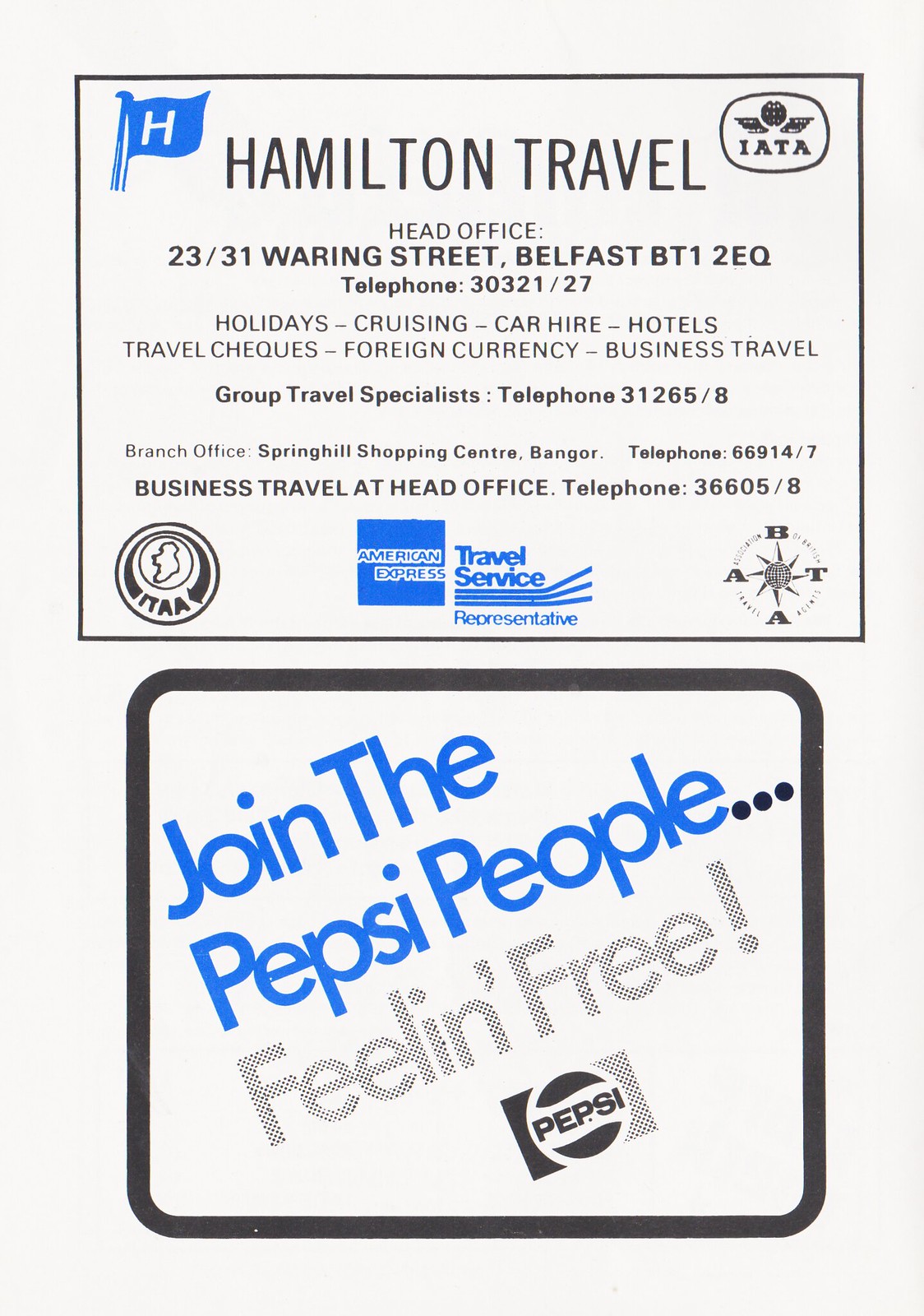The image presents a vintage black-and-white printed page from a publication in portrait orientation, embellished with spot color in blue. The top half features an advertisement for Hamilton Travel. At the very top, in black condensed sans-serif type, it reads "Hamilton Travel," with a small blue flag bearing a white "H" to the top left and the IATA logo in an ellipse on the top right. Below this, centered text identifies the company's head office at "23/31 Waring Street, Belfast BT1 2EQ." The ad includes various details such as telephone numbers, services like "Holidays, Cruising, Car Hire, Hotels," and highlights their expertise as a "Group Travel Specialist." Towards the bottom, there is an American Express Travel Service representative logo in blue, flanked by two additional black logos.

The bottom half of the page advertises Pepsi with a nearly square design. This ad features bold, dark blue lettering at an angle, stating "Join The Pepsi People..." followed by the phrase "Feeling Free!" in light gray. The iconic Pepsi logo and wordmark appear prominently at the bottom of the ad.